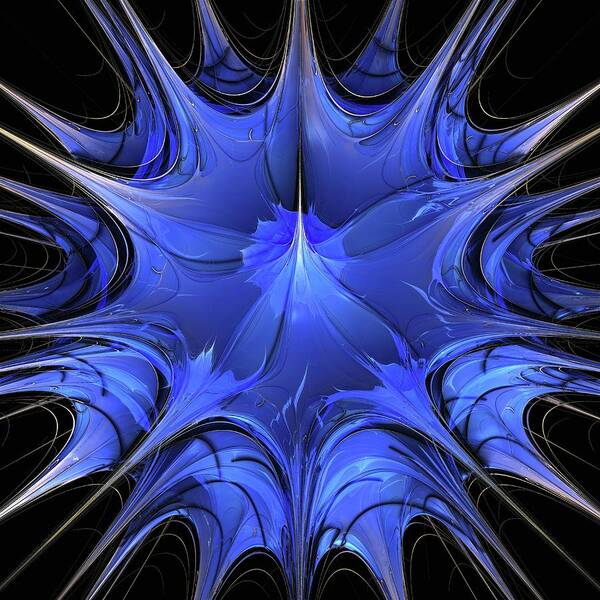This digital image features a complex and abstract design dominated by a deep, almost black background with undertones of dark blue. At the center of the image is a striking, spiky shape reminiscent of a spiked ball or a flower with sharp edges, extending outward in all directions. The central structure is digitally rendered in varying shades of blue and purple, interspersed with touches of white, creating a dynamic and textured appearance. The spiky form appears multi-layered and somewhat translucent, giving the impression of a flexible, fabric-like material being pulled and stretched. This layered effect adds depth and intricacy to the design. Overall, the image combines digital abstraction with a sense of movement and sharp detail, all encapsulated within the dark, deep blue backdrop.